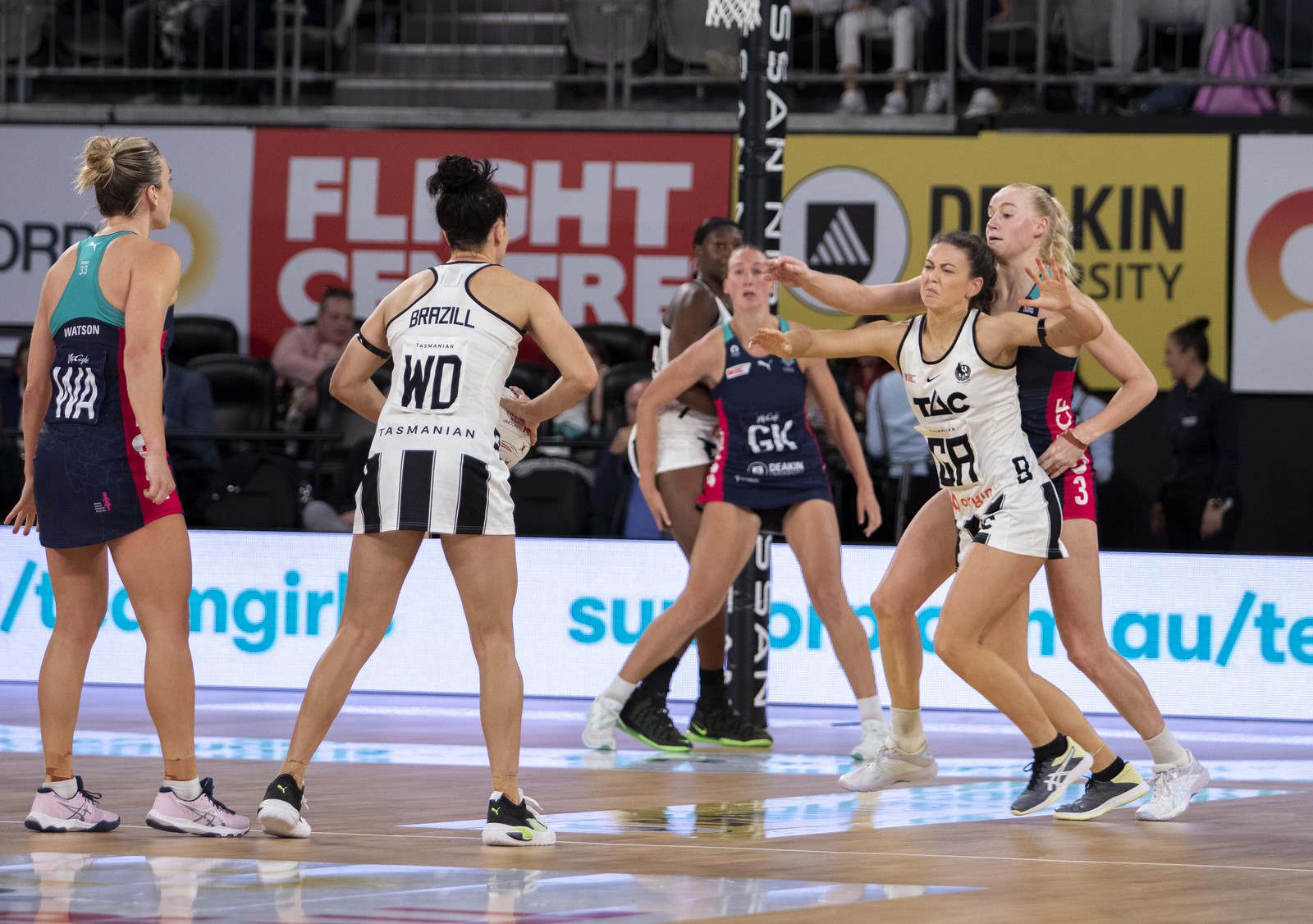The color photograph captures an intense indoor women's sports game, potentially a netball match, played on a wooden court decorated with various decals. In the foreground, six women are actively engaged in the game. The team wearing white jerseys with black and white skorts includes a player with "Brazil" and "WD" printed on the back of her jersey, indicating her defensive position. Another player on this team, facing the camera, has "TAC" on the front of her shirt. The opposing team is donned in blue jerseys with red and dark blue accents. The player in white holding a round ball suggests it is a netball, differentiating it from basketball. Surrounding the court, the background reveals two tiers of spectators alongside several advertisement signs, including "Flight Center" and references to a university. Visible in the scene is a black post of a basketball backboard with white print, hinting at the multifunctional use of the venue. The crowd, as well as a photographer, adds to the lively atmosphere of the match.